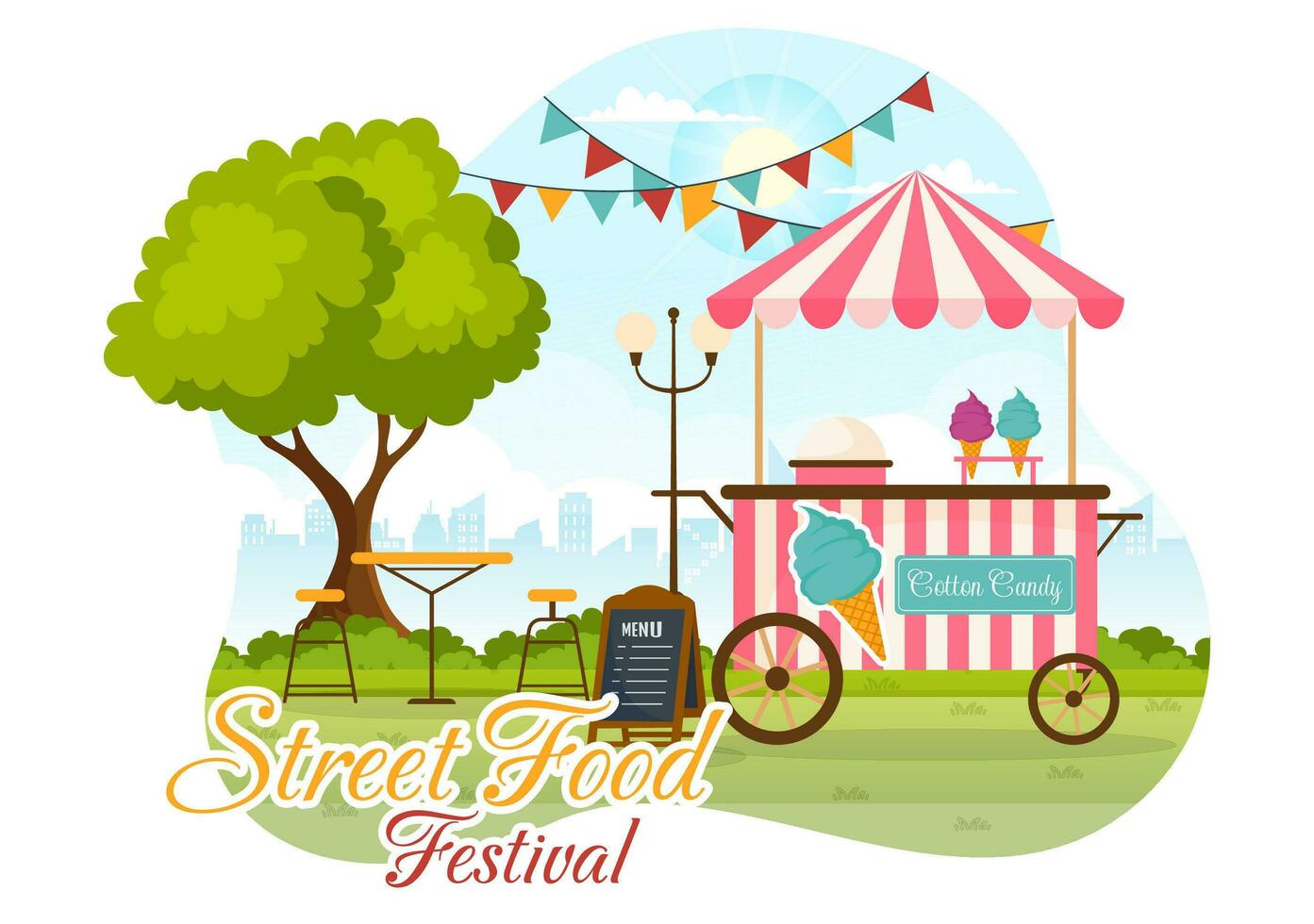This advertisement, characterized by a cartoonish aesthetic that could suggest AI generation, is wonderfully detailed and evocative. Against a clean, white backdrop, the bottom left corner features the text "Street Food Festival" in gold, with the word "festival" highlighted in red. Central to the image is an inviting scene: 

On the left side, a tree with a brown trunk and lush, green foliage stands over a picnic setting. The table, with a yellow surface and matching yellow seats, is accompanied by two brown-legged benches. This cozy picnic area rests on a patch of green grass. Just to the right, a brown sign prominently displays the word "Menu".

Further right, a whimsical cotton candy stand catches the eye. This portable food stand, adorned with pink and white stripes and a pink and white canopy, reads "Cotton Candy." Illustrations on the stand showcase a cone of light blue cotton candy, along with real cotton candy of various hues—light blue, purple, and others. In the background, the silhouette of a cityscape rises against a light blue sky, with an intriguing dark blue sun completing the scene.